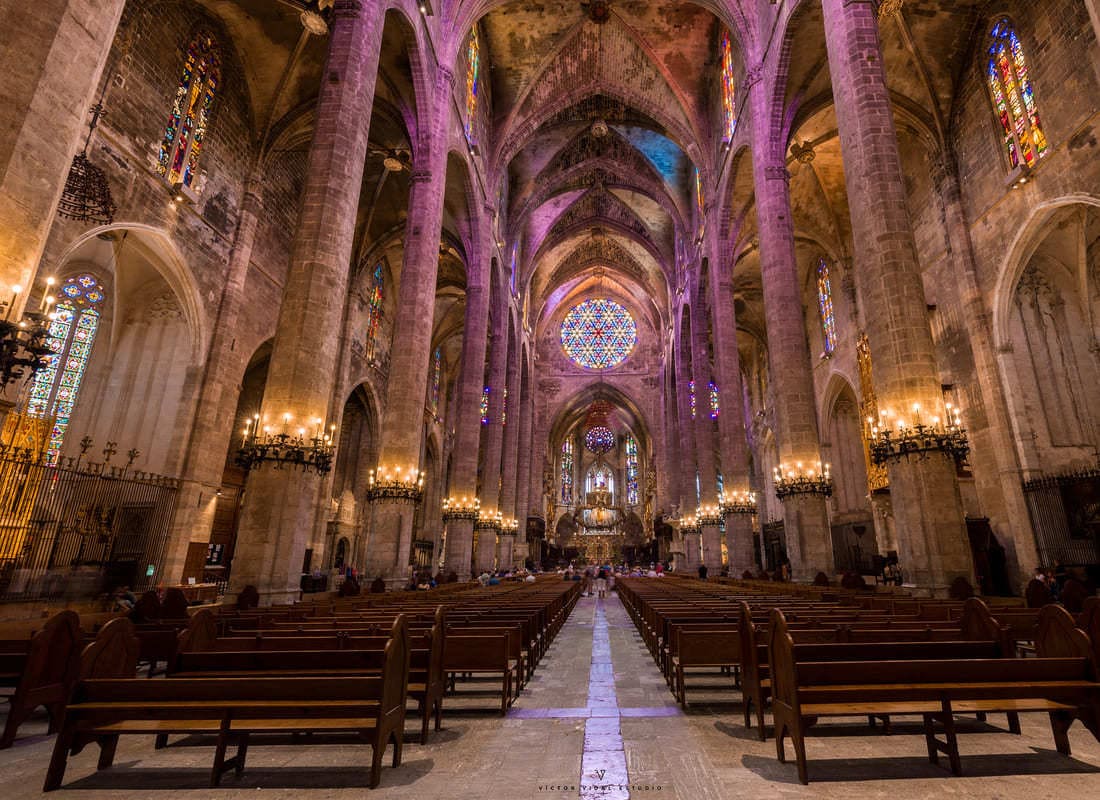This detailed image showcases the magnificent interior of a grand cathedral. The breathtaking view captures the immense height of the ceiling, soaring to approximately 50 to 70 feet, adorned with intricate stonework. Gigantic columns stretch from floor to roof, each graced with regal circles of candles that amplify the grandeur. The interior is predominantly dark brown, accentuating the elegance of the architecture. 

Lining the left and right sides of the cathedral are multiple rows of dark wooden pews, divided by a central tan floor that features a large cross. As the viewer stands at the very back entrance of the cathedral, the perspective leads towards the altar, which is flanked by an incredible array of stained-glass windows. To both sides, high, beautifully colored stained-glass windows allow light to cascade into the space, creating a mesmerizing display of colors.

At the far end of the hall, near the altar, there is an awe-inspiring, large circular stained-glass window, displaying an array of vivid yellows, blues, and reds. This intricate piece of artwork, almost half the size of the pulpit, is complemented by two narrow windows on either side. Below this stained-glass circle, a smaller, barely legible credit is inscribed. Occupying the far end of the pews and the center walkway, there are a few indistinct figures that appear to be people, contributing to the serene and solemn atmosphere of the cathedral.